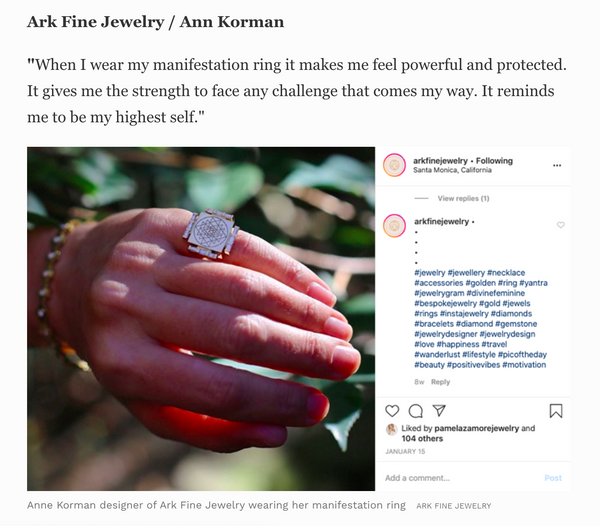The image is a social media post, likely from Instagram, showcasing fine jewelry by ARC Fine Jewelry and Ann Corman. At the top, in black letters, is the title "ARC Fine Jewelry / Ann Corman". Below the title are three left-aligned sentences in quotation marks: “When I wear my manifestation ring, it makes me feel powerful and protected. It gives me the strength to face any challenge that comes my way. It reminds me to be my highest self.” 

Underneath this text is a large square close-up photo of a person's left hand, adorned with a square-shaped, bulky ring on the pinky finger and a beaded bracelet on the wrist. The hand is extended towards the camera against a blurry outdoor background with green and brown colors, suggesting leaves and sticks. Below the image, there is a caption that reads: “Ann Corman, designer of ARC Fine Jewelry, wearing her manifestation ring. ARC Fine Jewelry.”

On the right side of the image, there is a column of information resembling a social media interface. It starts with a red circle and some black text, followed by a faint line and dash, and "view replies" in faint writing. Below that are more red circles with black text, lines of blue text likely representing hashtags such as #jewelry and #necklace, and a series of icons. The post also notes it is liked by a specific user and 104 others, along with a date, an option to add a comment, and a “post” button.